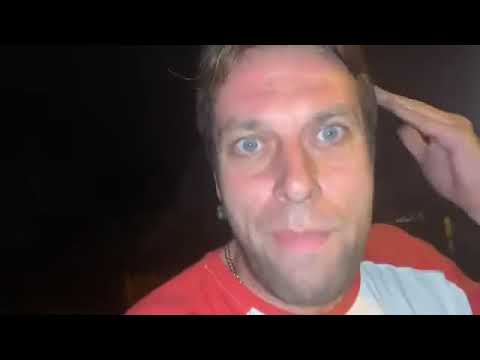The image is a selfie taken in a very dark setting, possibly outside at night, with the flash on, making the background completely black. The photo is framed with black borders at the top and bottom. The subject is a white male with light brown, slightly shaggy hair and bright blue eyes, staring intently into the camera. He appears to have a freshly shaved face with some stubble beginning to show. He is sporting a red and white raglan sleeve shirt and a partially visible gold chain tucked into his shirt. His left hand, with fingers close together, is touching his left temple. He has a slight side grin without showing his teeth. His face is well-illuminated, likely from the flash or the device used to take the photo, giving it a vlog-like appearance.